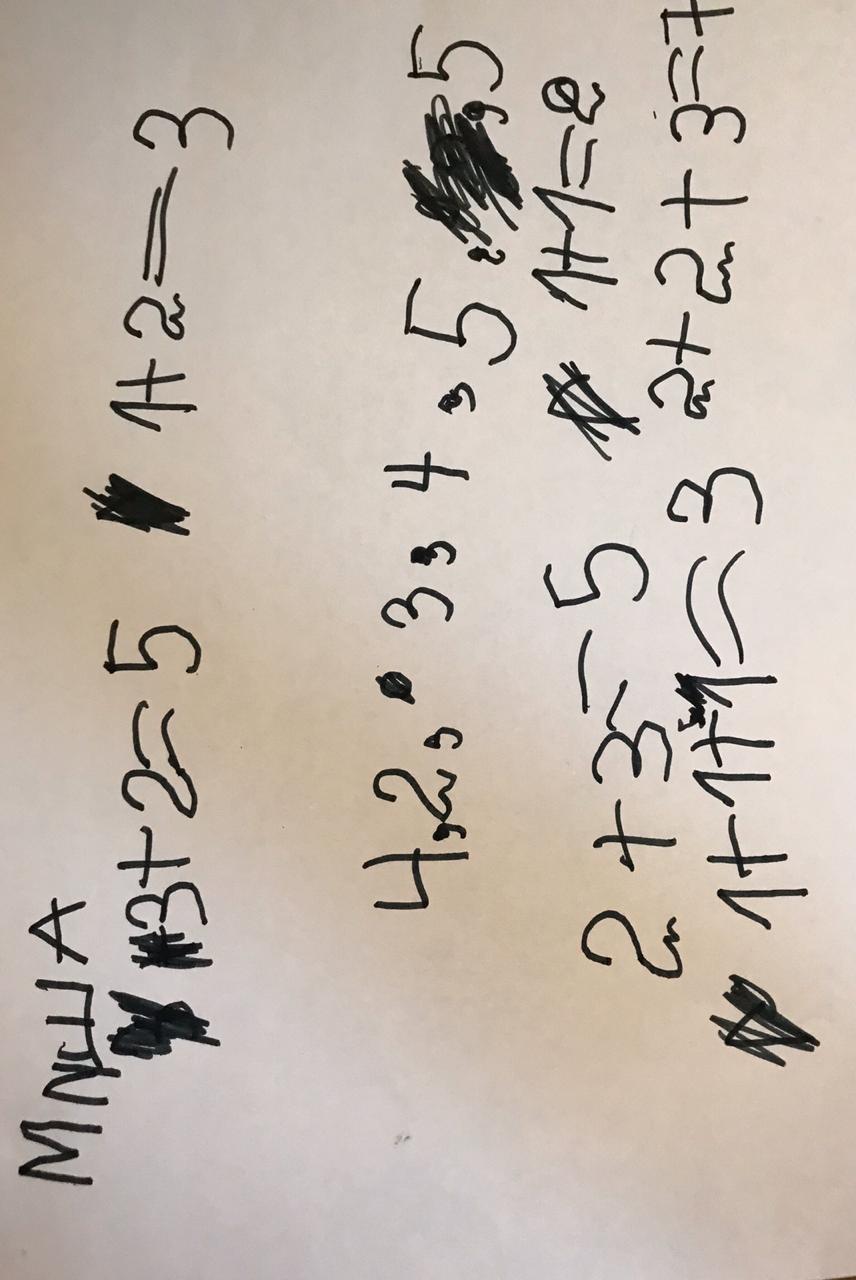The image depicts a long rectangular piece of white paper in portrait orientation, filled with what appears to be the early attempts at arithmetic and writing by a young child, possibly aged four to six. The paper is littered with numerous scratches and scribbles, characteristic of a child's handwriting. The arithmetic problems include simple sums such as "3 + 2 = 5," "1 + 2 = 3," and "2 + 3 = 5." The child has also attempted to count sequentially, marking numbers in a somewhat jumbled order: "4, 2, 3, 4, 5." In the bottom left corner of the paper, there are letters forming "MNWA," which suggests the child might be trying to spell their name. The entire scene captures the earnest, exploratory nature of a young learner engaging with early math and writing exercises.